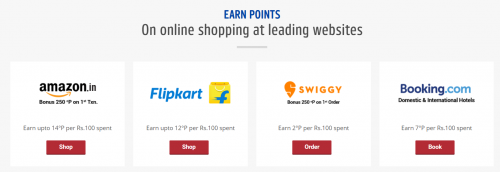This is a screenshot of a section from the EarnPoints website, which is dedicated to facilitating online shopping at leading websites. At the top of the section, "EarnPoints" is prominently displayed in blue, followed by the tagline "Online Shopping at Leading Websites" in grey. Below this header, there are four distinct white squares, each representing a different partner website. These squares feature the respective website logos along with the amount of points earned from shopping with each retailer. Each square also contains a red "Shop" button, inviting users to make purchases and earn points. The first website featured in this section is Amazon.in.